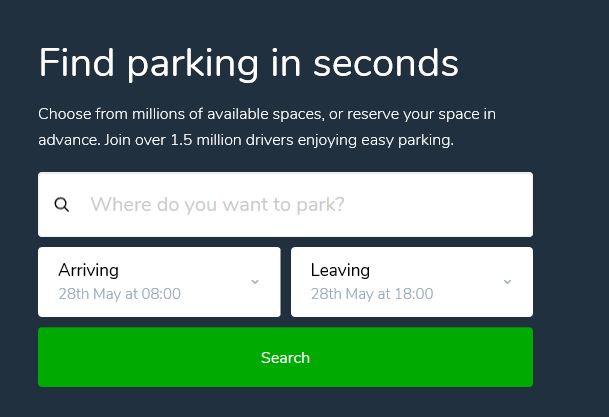The image features a black background with prominent white text at the top that reads, "Find parking in seconds." Below this, in smaller white text, it says, "Choose from millions of available spaces or reserve your space in advance. Over 1.5 million drivers enjoy easy parking."

Underneath this text, there is a white search bar with a magnifying glass icon on the left side. In the middle of the search bar, in gray text, it reads, "Where do you want to park?"

Beneath the search bar, there are two smaller rectangles. The left rectangle has text at the top in black that says, "Arriving," and below this, in gray text, it reads, "28th May at 08:00." On the far right side of this rectangle, there is a gray arrow pointing downwards.

The right rectangle mirrors this design, with black text at the top that reads, "Leaving," and gray text below stating, "28th May at 18:00." A gray arrow pointing downwards is also on the far right side of this rectangle.

At the bottom of the image, there is a large, dark green rectangle with the word "Search" written in white letters in the center.